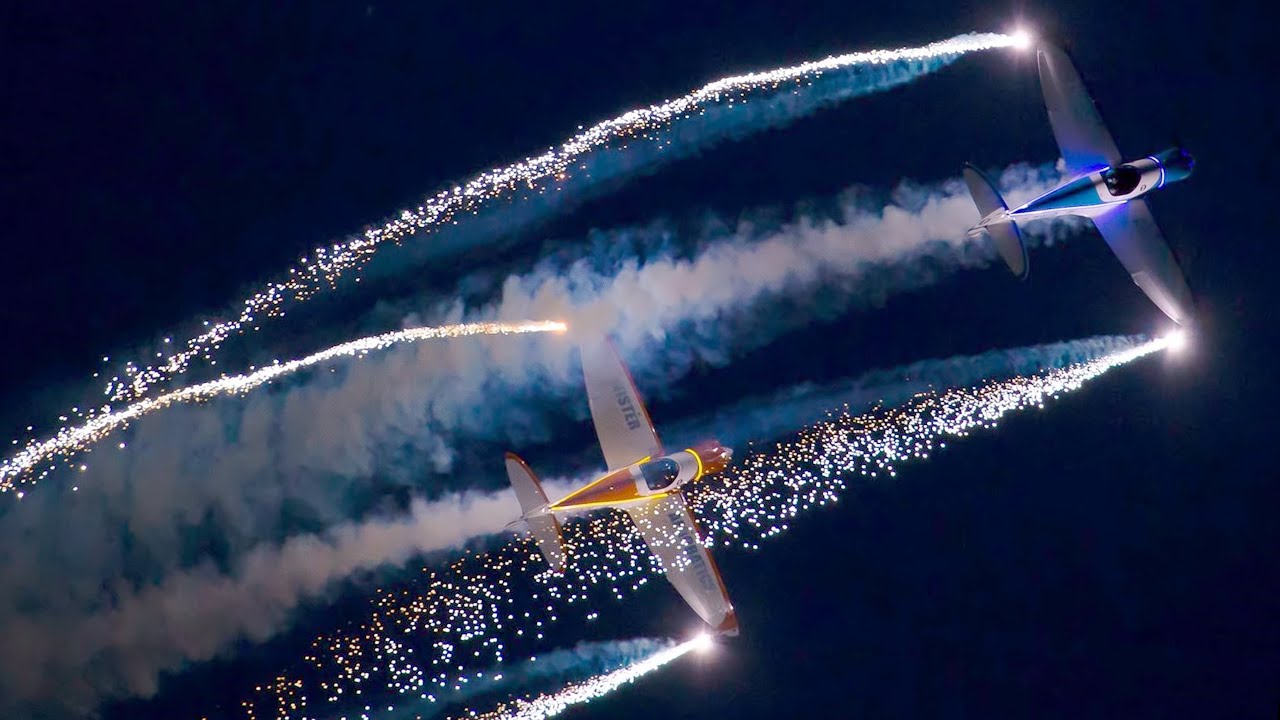The image captures a breathtaking night sky scene featuring two stunt planes engaging in an aerial display with fireworks and smoke. The plane positioned at the top right has a predominantly white body with striking blue accents at the nose and tail. This plane is adorned with bright lights at each wingtip, emitting cascading sparkles and a mix of blue and white smoke that beautifully trails behind it. The second plane, located at the bottom left of the image, showcases a white body accented with vibrant orange tips on its wings and tail. It too releases fireworks from its wingtips, accompanied by possible smoke trails. Both planes are captured in a dynamic, hard-turn maneuver, revealing only their top surfaces, with the illuminated and colorful smoke and sparkles accenting their acrobatic flight against the dark sky.